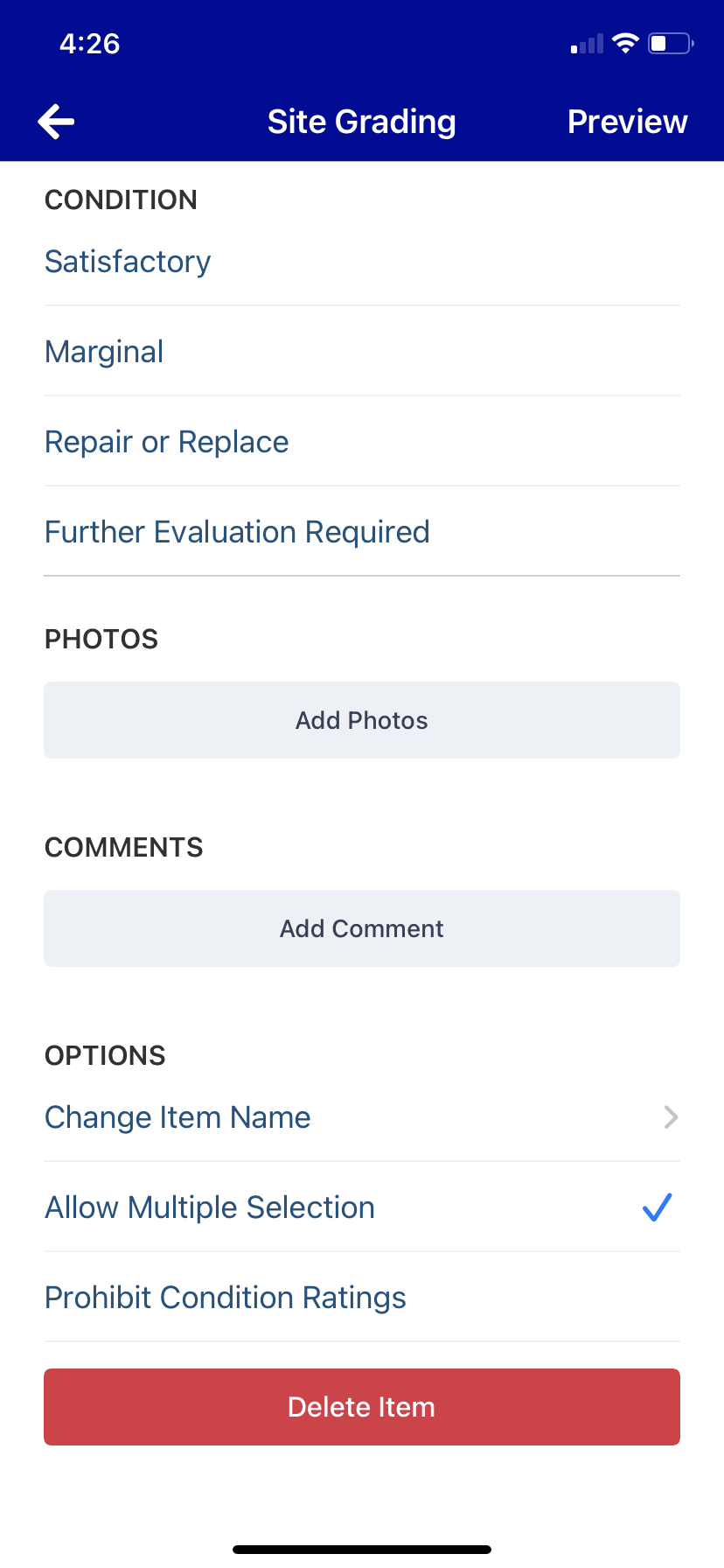In this image, a screenshot taken from a mobile device displays a detailed interface, likely from an application used for site grading or inspections. 

At the very top left corner of the screenshot, the time is indicated as "4:26," whereas the upper right corner shows a minimal cell reception with one bar out of four, a Wi-Fi icon with full strength, and a battery icon indicating approximately 35% charge remaining. The blue banner at the top center contains the text "SITE GRADING," flanked by a "Preview" button to its right, and a "Back" button to its left.

The main content of the screenshot features a white background. The top left corner displays a condition in black, all capital letters. Directly beneath this, the word "SATISFACTORY" appears in blue text, followed by a line. Below that, subsequent categories are listed in black text: "MARGINAL," "REPAIR OR REPLACE," and "FURTHER EVALUATION REQUIRED," each separated by a line and capitalized.

Further down, a section labeled "PHOTOS" in black, all capital letters is displayed, adjacent to a gray button featuring black text that reads "Add Photos." Below this section, the word "COMMENTS" is written in all capitals, followed by a gray box suggesting users to "Add Comment."

The "OPTIONS" section in all capital letters follows, displaying more blue text options: "Change Item Name" with an arrow pointing to the right, "Allow Multiple Selection" with a check mark, and "Prohibit Condition Ratings." At the bottom, a red "Delete Item" button concludes the interface.

This screenshot meticulously details an app interface for documenting and grading site conditions, presenting various options and functionalities in a neat and organized manner.